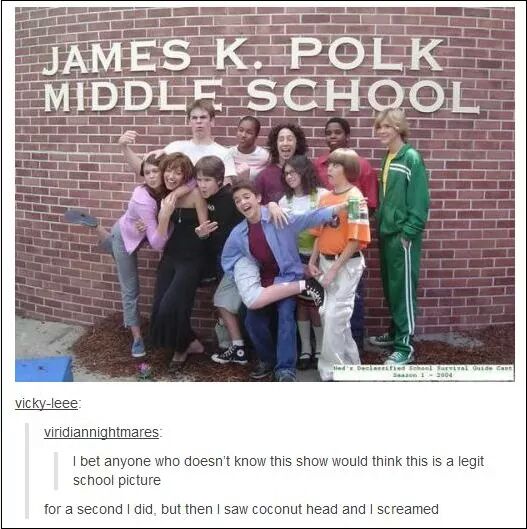This color photograph, ostensibly made for a web page, is bordered by a thin black line and features Vicki Lee, underlined, with Viridian Nightmares written below it in black text. The image captures a group of middle school-aged children and their teacher posing against a red brick wall with the inscription "James K. Polk Middle School" in large white uppercase font. The children, numbering more than ten, are arranged in two rows, wearing casual clothes like tracksuits, jeans, and shirts, and appear to be laughing and enjoying each other’s company. They exhibit playful gestures, with one student standing on one foot and a girl in a pink sweater hugging another girl in black. Notably, a student with a distinctive bowl cut, nicknamed Coconut Head, is visible, which ties into the humorous caption beneath the photo: "I bet anyone who doesn't know this show would think it's a legit school picture. For a second I did, but then I saw Coconut Head and screamed." At the very bottom, on the right corner, there is a white box with illegible tiny black text, and in the bottom left-hand corner, there's a blue square object. The reddish area under their feet seems like it might be chipped paint from the wall.